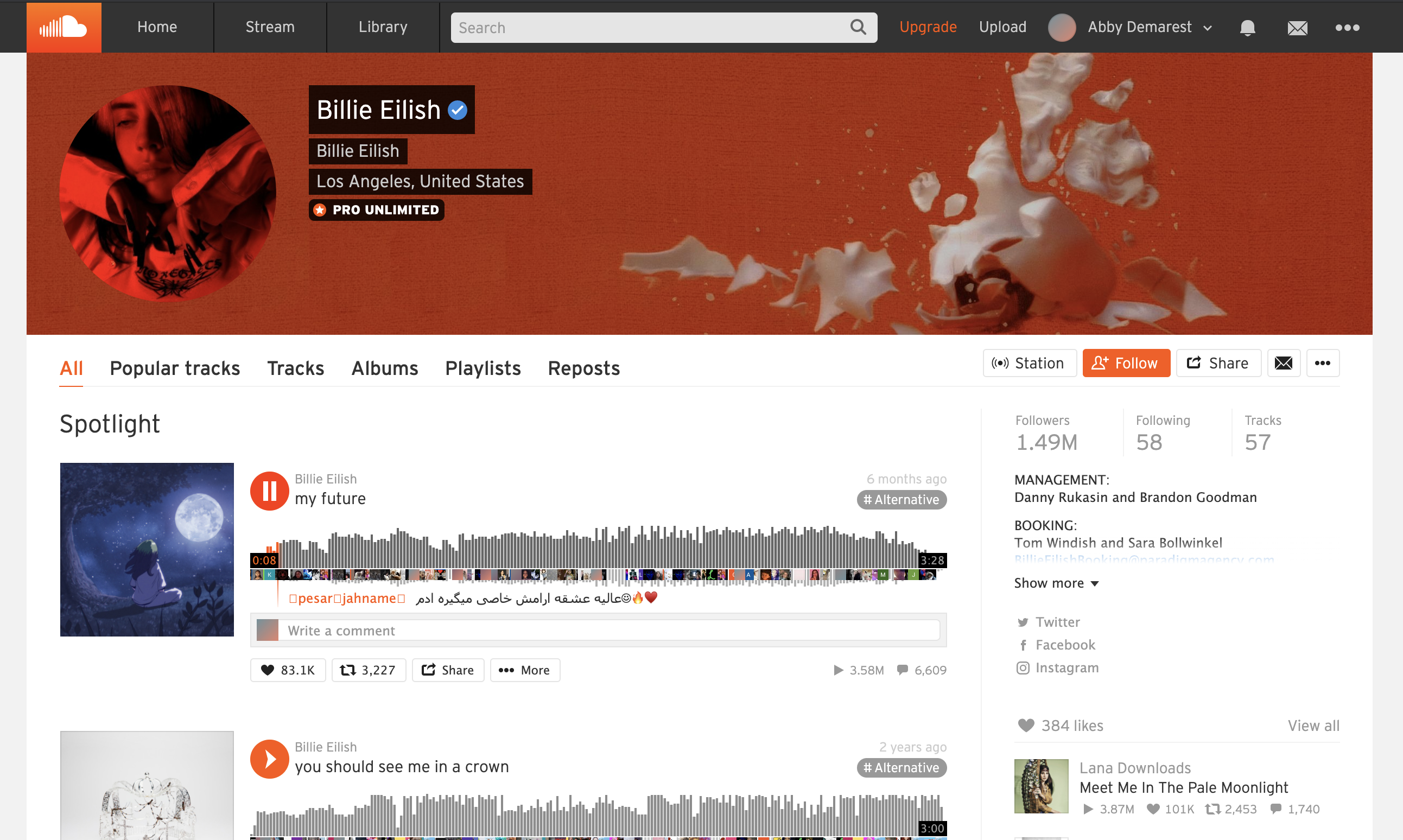The image depicts a website interface with a sleek and user-friendly design. At the very top, there's a thin black banner featuring an orange square with a white cloud icon inside it. Within this black header, the text "Home Stream Library" is written in white.

Just below the banner, there is a large white search bar with a black magnifying glass icon at the end, accompanied by an orange button labeled "Upgrade". Further along, in white text, it displays "Upload", "Abby Demarest", and icons for a bell, an envelope, and three vertical white dots.

Below this header section, the background transitions to an orange hue, showcasing a circular user or artist image. The text beside the image reads "Billie Eilish, Billie Eilish, Los Angeles, United States, Pro Unlimited".

Further down the page, tabs are arranged for different categories including "All", "Popular Tracks", "Tracks", "Albums", "Playlists", and "Reposts". Below these tabs, there's an option for "Station" and "Hello Share".

The page prominently displays different albums by Billie Eilish, highlighting titles such as "My Future" and "You Should See Me In A Crown".